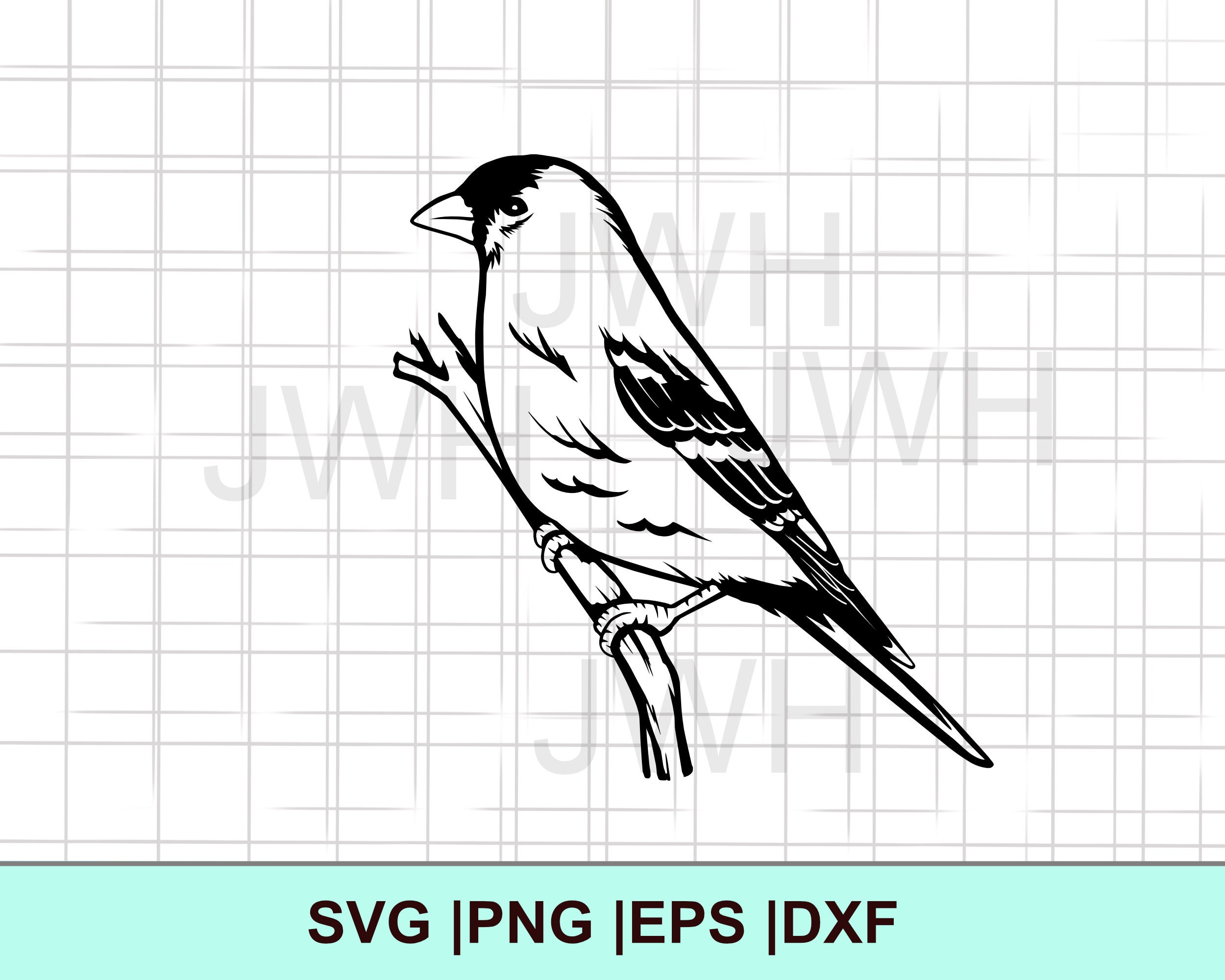This stock-like graphic features a black and white illustration of a bird, resembling a finch or sparrow, perched on a wooden branch. The bird, centrally positioned and facing left, is rendered in a hand-drawn style, although it could be digitally created. The head of the bird is shaded with black, and its feathers and tail exhibit darker tones. The background of the image is covered in a pale gray grid and marked with a repetitive watermark labeled "JWH". At the bottom of the graphic, a turquoise strip displays the text "SVG, PNG, EPS, DXF" in black font, indicating the available file types for download.